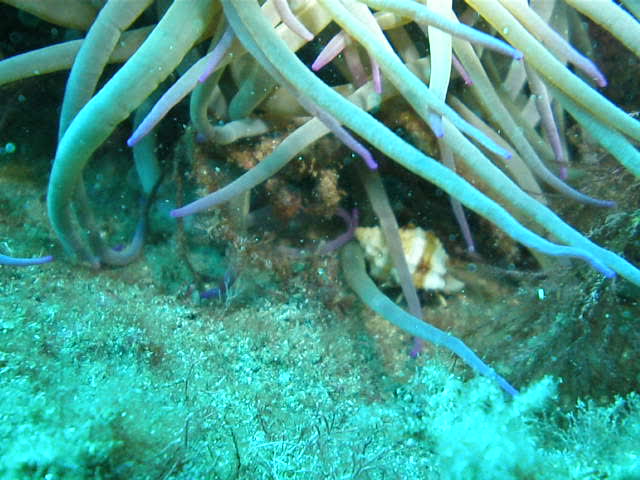The image depicts an underwater scene showcasing the seafloor teeming with diverse aquatic plant life. Dominating the scene is a striking underwater plant, characterized by its long, wiry tentacles resembling a mix between vegetable roots and fin tree roots. These tentacles, emerging from the top of the frame and cascading down, exhibit a captivating gradient from green to light green, and taper off into hues of pink and purple. Nestled among this verdant display is a small shell, which appears to house a creature — likely a crab — with visible legs peeking out. The backdrop of the image includes a dense carpet of algae-like plants in lighter shades of green, enveloping the floor in a drab, mellow greenish-blue ambiance reminiscent of an underwater meadow. The entire scene conveys a sense of serene, otherworldly beauty through its vibrant yet subdued color palette.